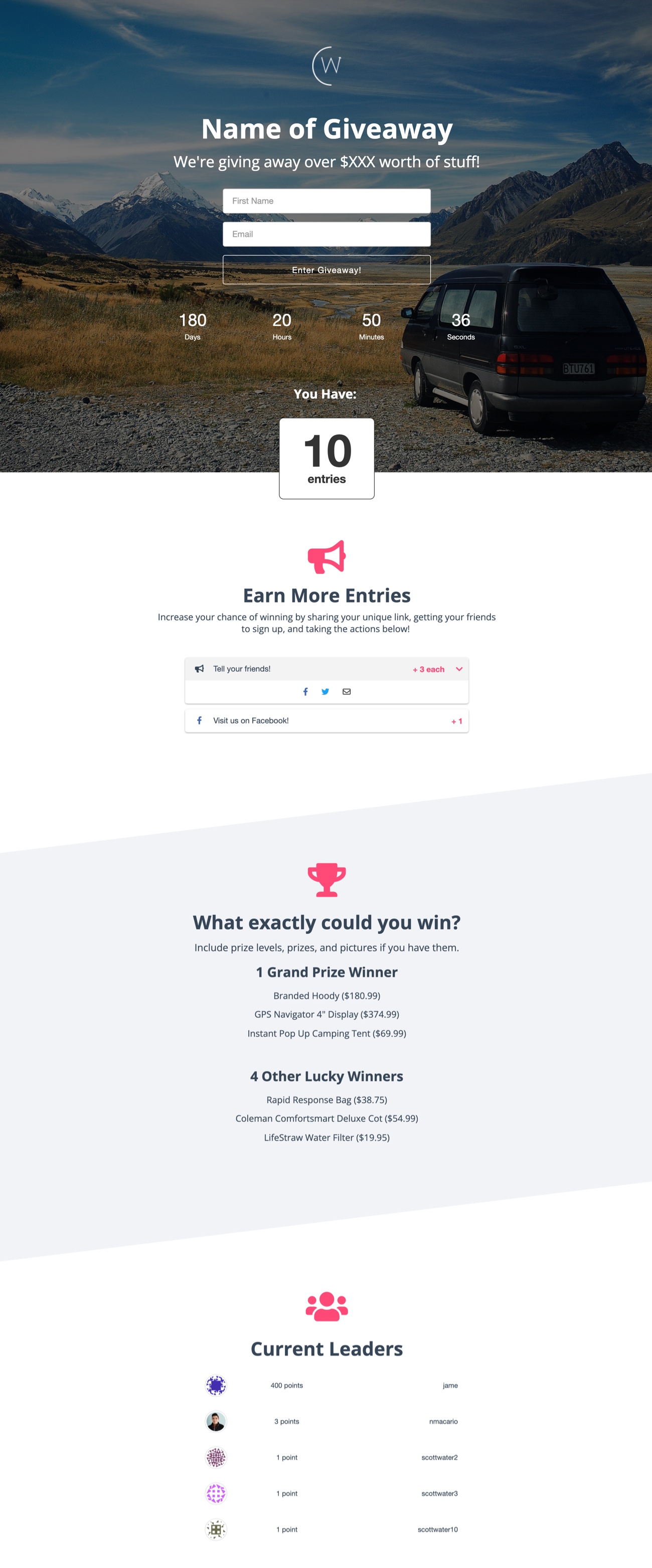A detailed screen capture of a web page features a dominant, large, horizontal image of a van. The dark-colored van is positioned in the lower right-hand corner, facing outward toward a breathtaking panoramic view of snow-capped mountains and desert grasses. At the top of the image, in bold white letters, it says "Name of Giveaway" within a white semicircle featuring a white 'W' in the center. Below this is a proclamation: "We're giving away over $XXX worth of stuff."

Underneath this slogan, there are two white text boxes, inviting users to participate by entering their details. The first text box is labeled "First Name," and the second one is labeled "Email." A button below these fields, with white lettering, prompts users to "Enter Giveaway."

The countdown timer below this reads: "180 days, 20 hours, 50 minutes, and 36 seconds to go." It is accompanied by a bold message in white text: "You Have," followed by a black box stating "10 entries."

Prominently beneath this is a red megaphone icon, which provides instructions for earning additional entries. It encourages participants to increase their chances of winning by sharing a unique link, getting friends to sign up, and performing specified actions. The initial actions offered are "Tell your friends" and "Visit Facebook."

Following this, on a light gray background, is a red Loving Cup icon. A bold label beneath this icon asks, "What Exactly Could You Win?" It indicates one grand prize winner and four additional lucky winners.

At the very bottom of the page, an icon of a human figure with sweat drops emanating from both sides is displayed. Beneath it, in black text, it reads "Current Leaders," listing the top five participants, with the leading person having amassed 400 points.